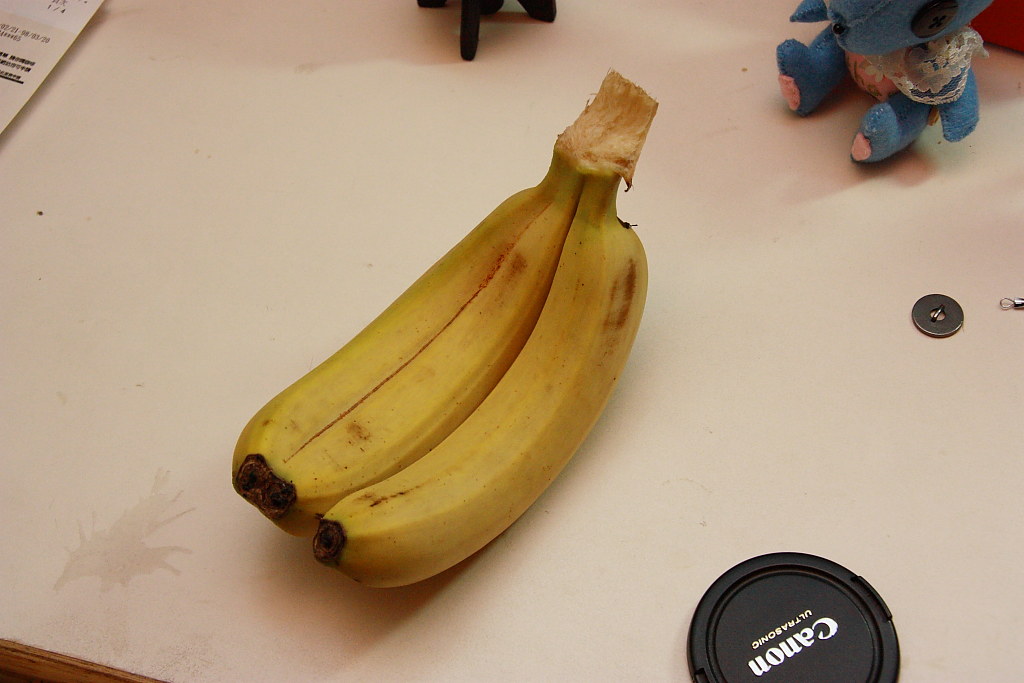In this detailed image, the top of a white table serves as the background. Centrally placed on the table are three vibrant yellow bananas, still connected at the stem and positioned side by side. On the bottom right corner of the table lies a black, circular plastic lens cap, emblazoned with the brand name "Canon" in white text, though the writing appears upside down in the image.

Towards the top right-hand corner, a small blue plush stuffed animal is partially visible. This toy resembles a bear, with pink paws and is dressed in pink clothes adorned with a delicate white lace collar. The bear's eyes are represented by black buttons, adding a charming touch. Slightly below the plush toy, there is a small circular silver object with a hole in the center, resembling a coin or a washer.

In a position just above the bananas, a small black stand with four legs can be seen, adding to the assortment of items on the table. Additionally, on the left side of the image, the edge of a white piece of paper with black typed text is visible, possibly a receipt or a document. The diverse objects scattered across the white table create an intriguing still life composition filled with varied textures and colors.